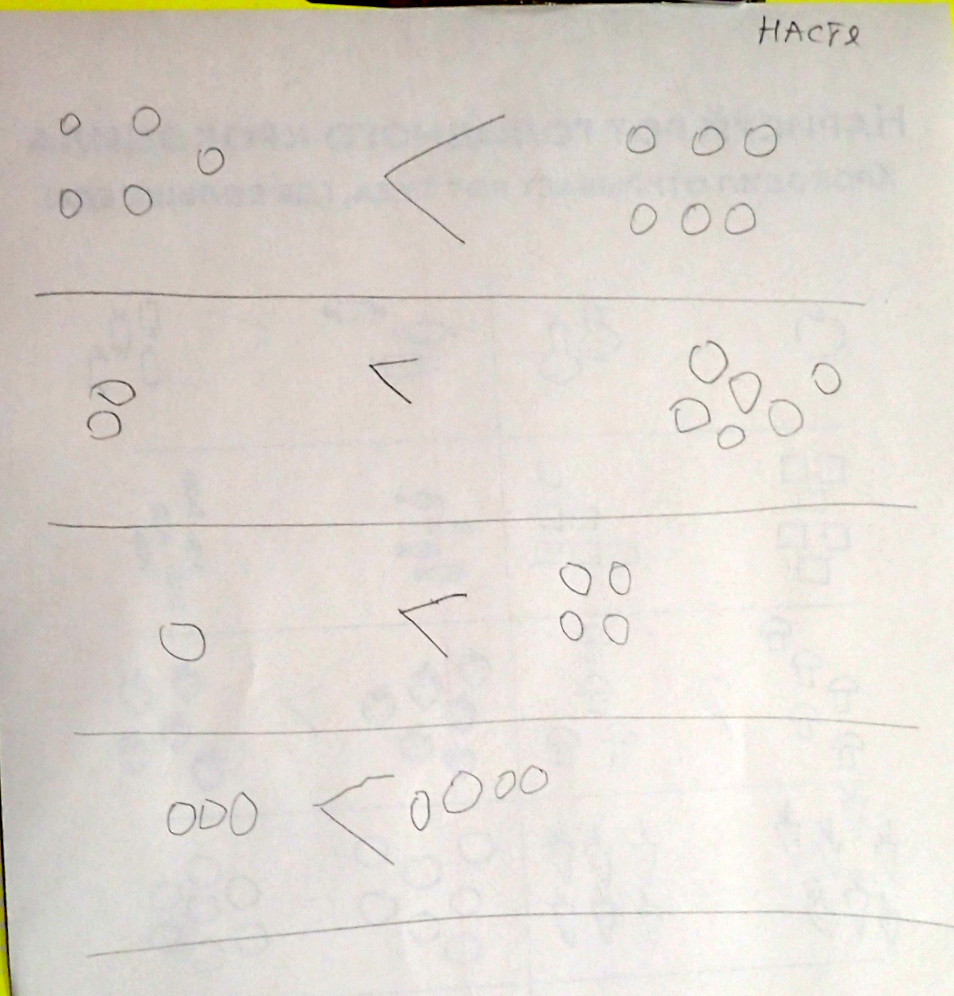A white piece of paper is photographed. In the upper right corner, it features the word "H-A-C-T-E" (hacked) written prominently. On one area of the paper, there are six circles arranged in a specific pattern with a "greater than" arrow symbol (>) pointing towards five more circles. Proceeding along the left-hand side of the paper, there is a black line accompanied by various groupings of circles connected by "greater than" arrows. In sequence, the black line starts with two circles pointing towards six circles, then a single circle pointing towards four circles. Further down, the line shows three circles pointing towards four circles.

The paper appears to have other figures and shapes faintly visible through it. Notably, in the middle-right section, there are square shapes, and on the top portion, there are backward letters starting with "H" and "A," followed by an "R," though the rest of the letters and circles are not entirely legible.